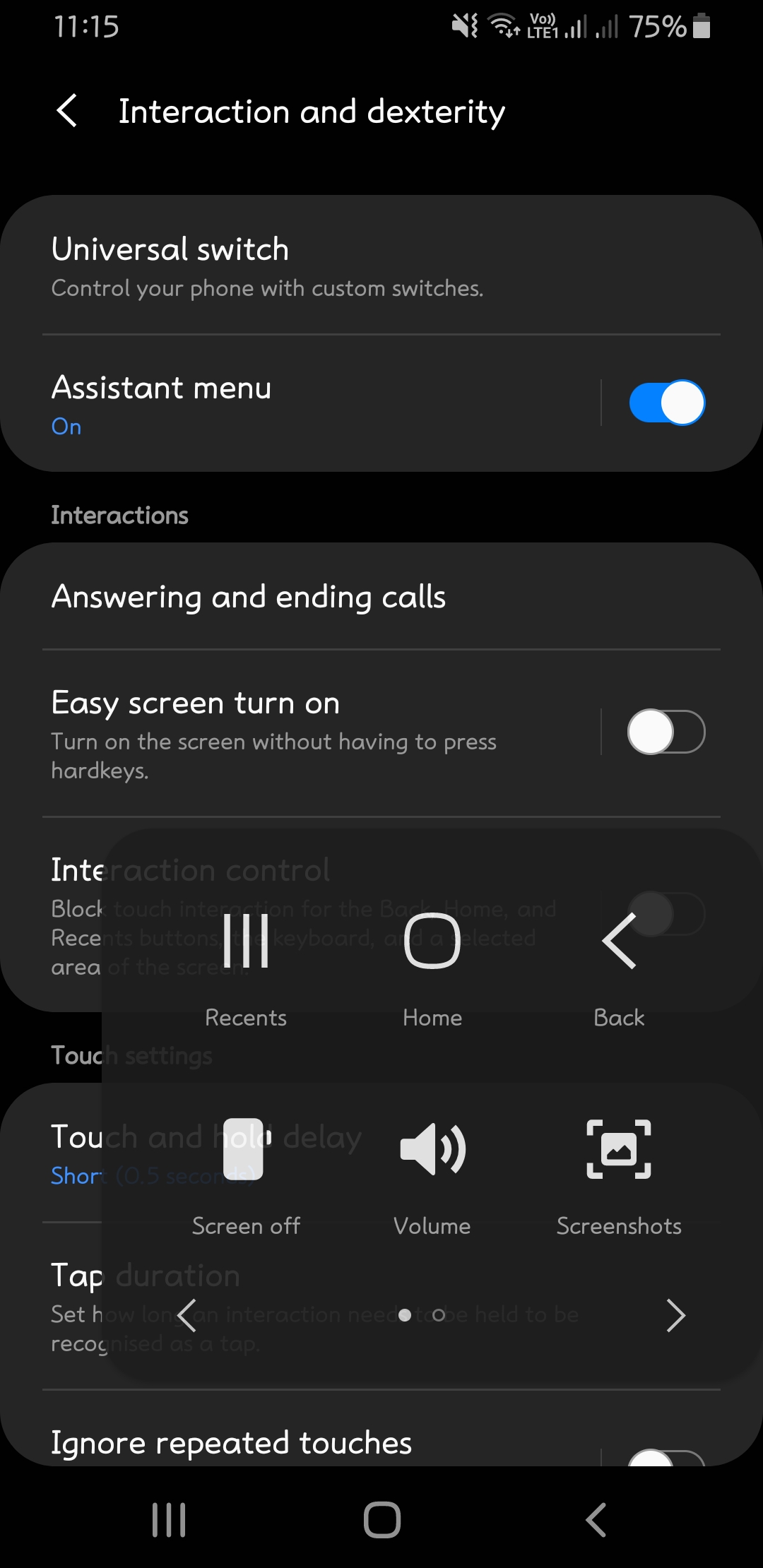In this image, we are viewing a web page titled "Interaction and Dexterity," which appears to be related to phone call functionalities. At the top left, the time is displayed as 11:15, while the top right shows the battery level at 75%. Directly beneath the "Interaction and Dexterity" header, there is an option labeled "Universal Switch," which indicates the ability to control the phone using custom switches. Below that is an option to toggle the "Assistant Menu," which is currently turned on.

The page continues with sections such as "Answering and Ending Calls" and "Easy Screen Turn Off," each accompanied by a switch knob located to the right. The "Easy Screen Turn Off" option is currently turned off. 

A prominent overlay on the lower part of the screen shows buttons labeled "Recent," "Home," "Back," along with options for "Screen Off," "Volume," and "Screenshots," which obscure some of the underlying settings. At the very bottom of the visible area, there is an option labeled "Ignore Repeated Touches," which is currently turned off as well. This detailed interface allows for extensive customization of interaction and dexterity settings on the device.